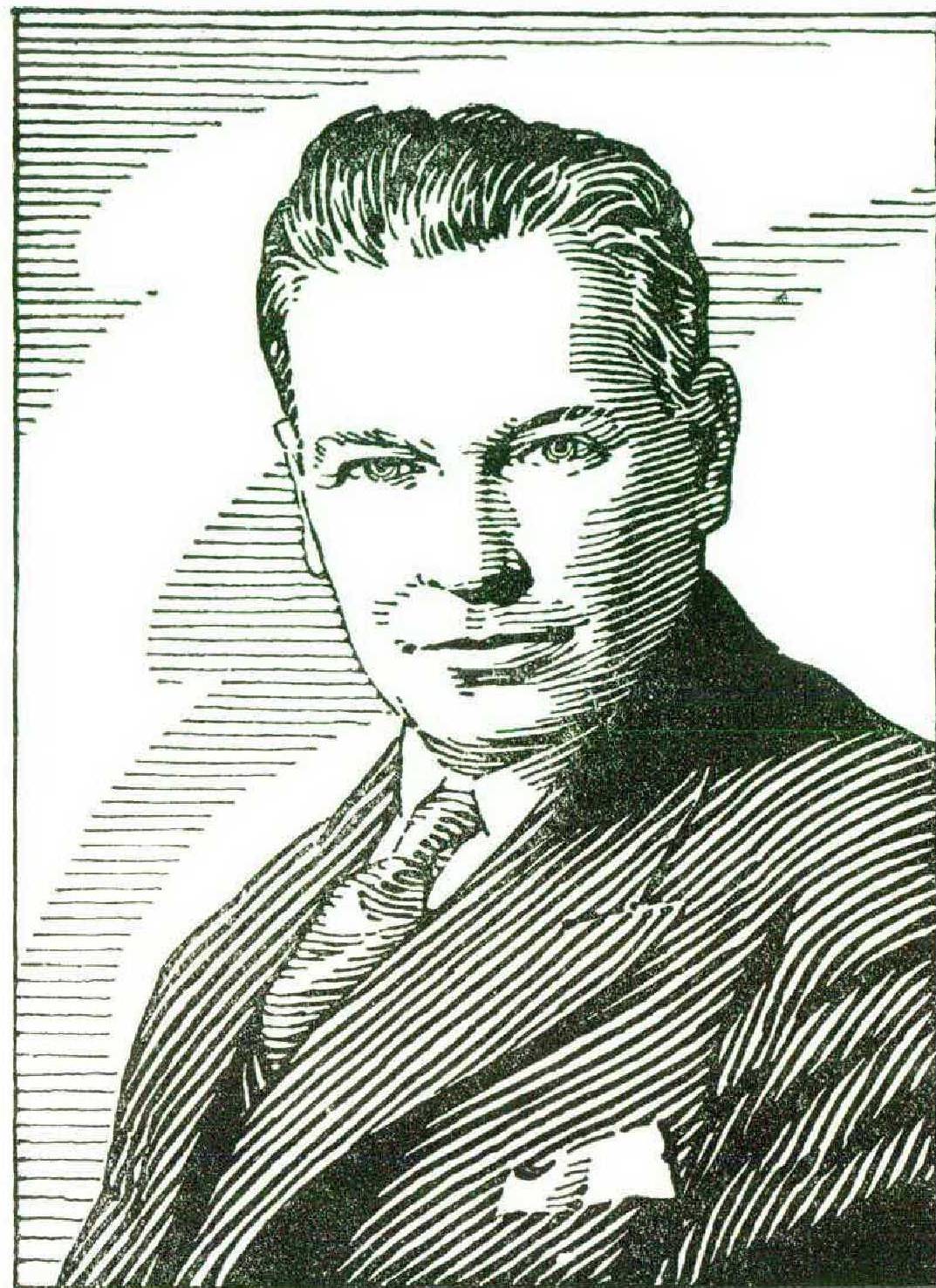This black-and-white illustration, reminiscent of the style found in the Wall Street Journal or on a dollar bill, portrays a man with precise and exquisite detail. He has short, wavy hair that's neatly combed back and wears a pinstripe suit with a matching pinstripe tie. A handkerchief is neatly tucked into his lapel pocket. His face, devoid of any beard or mustache, bears a slight, pleasant smile, and he gazes directly at the viewer despite his head being slightly turned to the left. The background, composed of line art resembling clouds, enhances the intricate shading and texturing of the drawing, giving it a realistic photographic quality. The entire composition is set within a bordered frame, highlighting the meticulous craftsmanship of the artist.